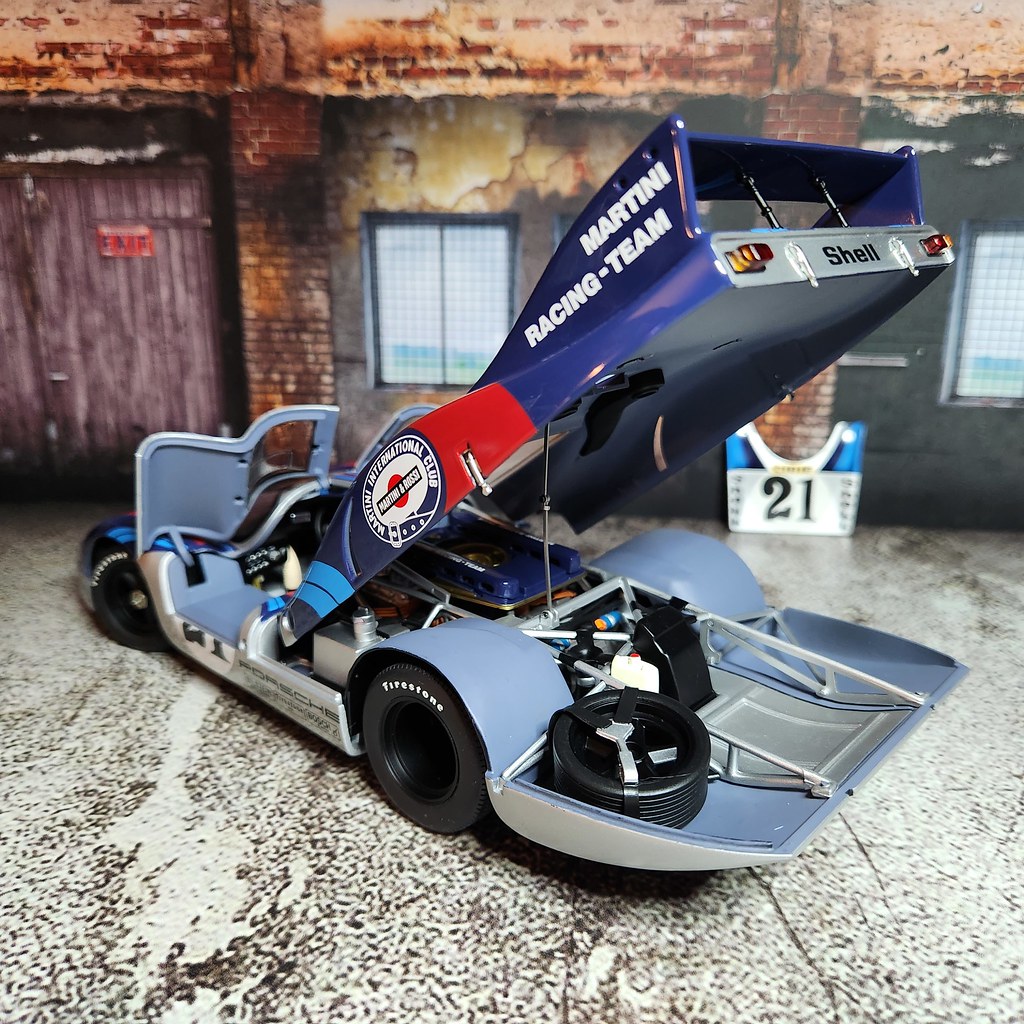The image showcases a highly detailed scale model of a racing car set within a meticulously crafted garage scene. The model car, designed with realistic features, has its body lifted to reveal a faux engine and a spare tire underneath. The body, a mix of navy blue and cobalt blue with red accents, is propped up on a tiny metal wire to exhibit the intricacies of the car's underside. The car's cockpit, with a black steering wheel and silver-painted knobs, is visible as the front is also lifted. The chassis is composed of blue and gray metal, and the black wheels have white 'Firestone' lettering.

The vehicle is adorned with the 'Martini Racing Team' logo on the elevated upper fin, visibly in white lettering, and bears another red logo with a white circle featuring text too small to discern clearly. Additional text 'Team International' is present on the side. The chassis, equipped with four wheels, is situated on a heavily textured flat surface mimicking a concrete floor with brown pits.

The backdrop of the scene is a printed representation of a warehouse wall, designed to resemble red brick with visible flaking. Windows are indicated in the background along with a wooden door that complements the slightly dilapidated aesthetic. The setting includes a numbered stand with '21' inscribed on it, reinforcing the illusion of a garage environment where the model car is presumably being worked on or displayed.